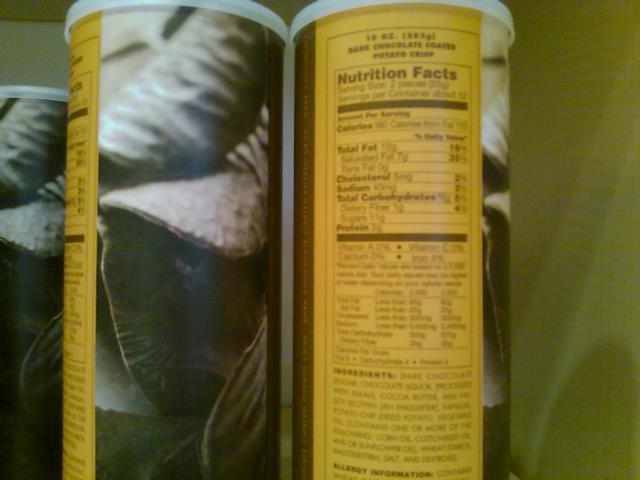The image features two cylindrical food product packages positioned centrally against a white wall, creating a backdrop with visible shadows cast by the packages. Each package is tall, with a white lid. The packaging on one of the cans displays an image, suggesting it is part of the product's branding. The second package prominently features a nutrition label.

The nutrition label is set against a yellow background with brown-colored text. It details the product as "Potato Crisps" and specifies the net weight of the contents as 10 ounces. The label includes comprehensive nutritional information, listing values for total fat, cholesterol, and sodium, among other nutritional facts. Additionally, it provides a list of ingredients and allergy information. The overall setup and product presentation indicate it is an edible item, specifically a savory snack.